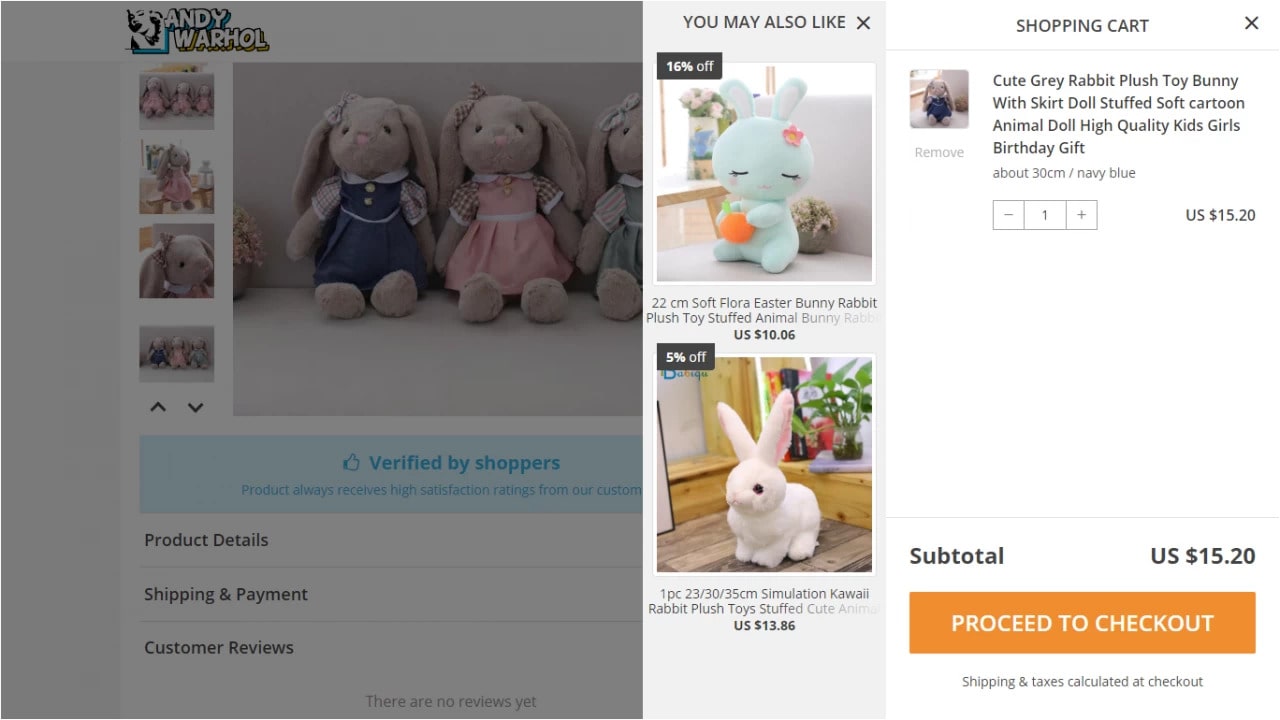The image depicts a section of a shopping website focused on Andy Warhol-themed merchandise. At the top left of the screen, "Andy Warhol" is prominently displayed. Below this title, thumbnail images of products for sale are arranged vertically. Highlighted among these products are three uniquely dressed bunny dolls, each adorned with a plaid hair ribbon and a pink nose. These bunnies are clad in different dresses and feature plush, bear-like feet. 

To the right of these thumbnails is a product section that includes customer interaction options. It mentions “Verified by Shoppers,” indicating that the product consistently receives high satisfaction ratings, although part of the text is cut off. Additional tabs below this provide further details under headings such as "Product Details," "Shipping and Payment," and "Customer Reviews." Notably, there are no customer reviews yet.

Adjacent to this, an area titled “You May Also Like” showcases other related products. One featured product is a 22-centimeter soft plush toy of an Easter bunny holding a carrot, offered at a discounted price of $10.06 (16% off). Another item displayed is a more realistic plush bunny with long ears, available in various sizes (23cm, 30cm, 35cm) and priced at $13.86 with a 5% discount.

On the far right of the page, the Shopping Cart section lists an item described as a "Cute gray rabbit plush toy bunny with skirt doll stuffed soft cartoon animal doll," ideal as a high-quality birthday gift for kids. This particular bunny is about 30 centimeters tall and is priced at $15.20. The subtotal for the cart is $15.20, with a prompt to proceed to checkout, while noting that shipping and taxes will be calculated at that stage.